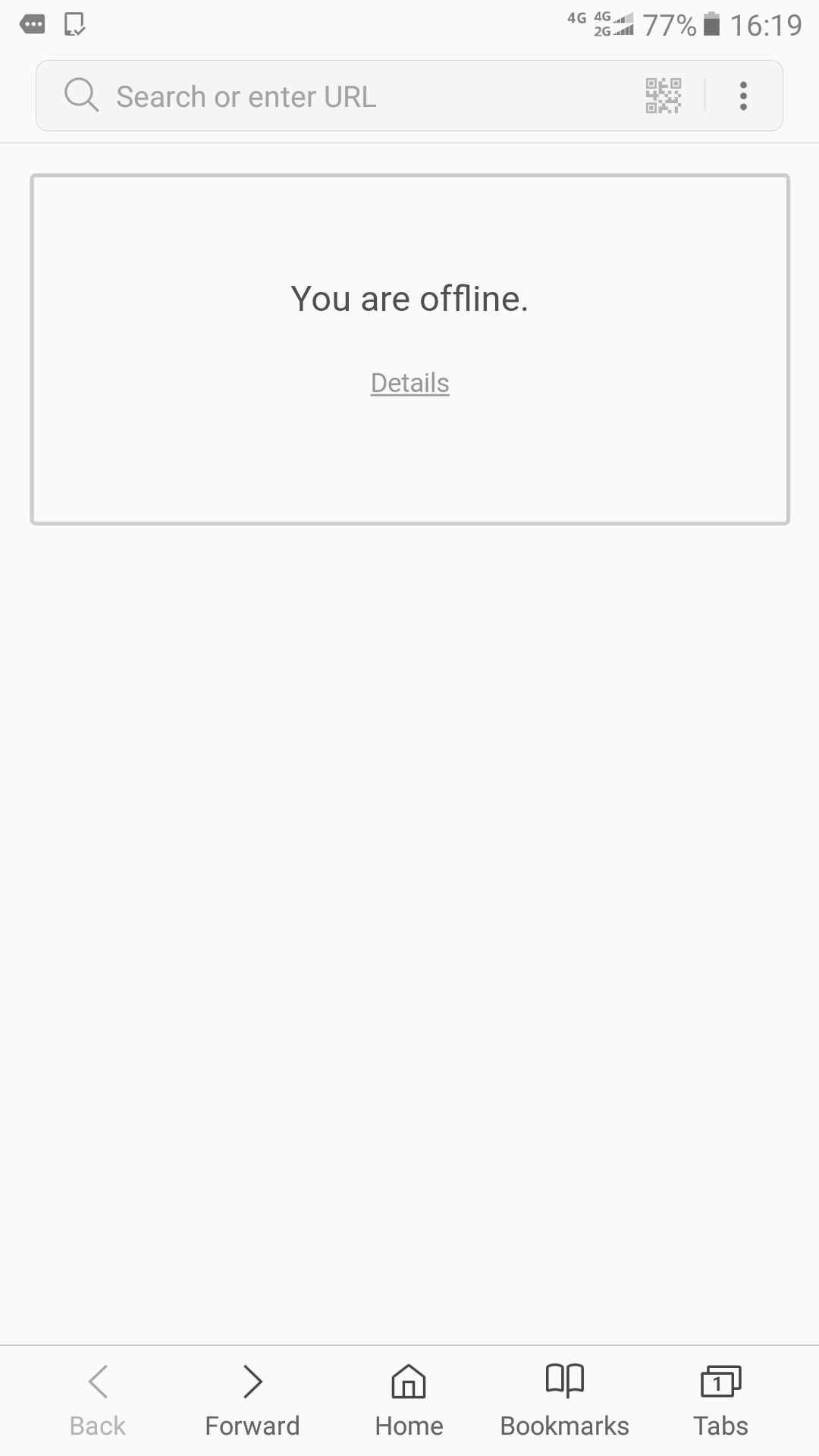The image depicts a distinctive white cell phone with a gray tag featuring three white dots located in the upper left-hand corner. The device displays "4G," indicating a weak signal compared to the more prevalent 2G network. The battery level is at 77%, and the time is shown as 16:19 (4:19 PM in military time). 

At the top of the screen, there is an empty search bar, followed by a large rectangular box in the center with the message "You are offline." There is an option to click on "Details" beneath this status message. It appears that the user has been attempting to download something via the 4G network, but the lack of a strong connection has hindered this process.

At the bottom of the screen are the standard navigation buttons: back, forward, home, bookmarks. Multiple tabs seem to be open, but due to the offline status, their contents are currently inaccessible.